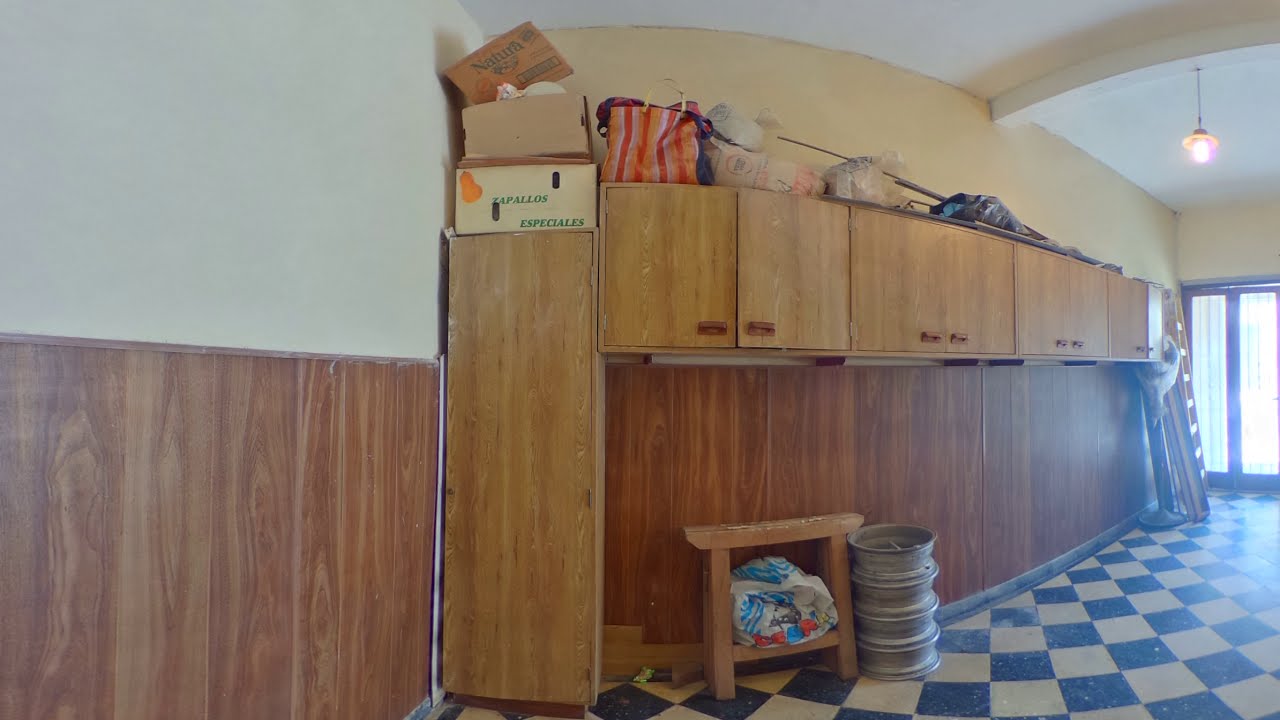This photograph captures an empty, old room that appears to have been used for storage. The checkered black-and-white flooring is worn and dirty, showing years of use. Along the right side of the room, a window with a cherry wood frame features two panels divided down the middle. Directly below this window, the bottom half of the wall is covered in dark wood paneling, transitioning to lighter wood cabinets with matching cabinet doors. These cabinets stretch from right to left and are cluttered with various items, including boxes labeled "Apollos Especiales" adorned with an orange design, as well as tools, bags, and other random objects. Visible on top of these cabinets are also boxes marked "Zappalos Especales" and "Natura." Towards the far left, the top half of the wall is a blank white, which contrasts with the dark wood paneling below. Additional storage elements within the room include a small stool next to a cylindrical metal object and a stack of about four tire rims. In the far right of the image, a glass doorway lets in bright sunlight, illuminating the space and suggesting it's daytime.